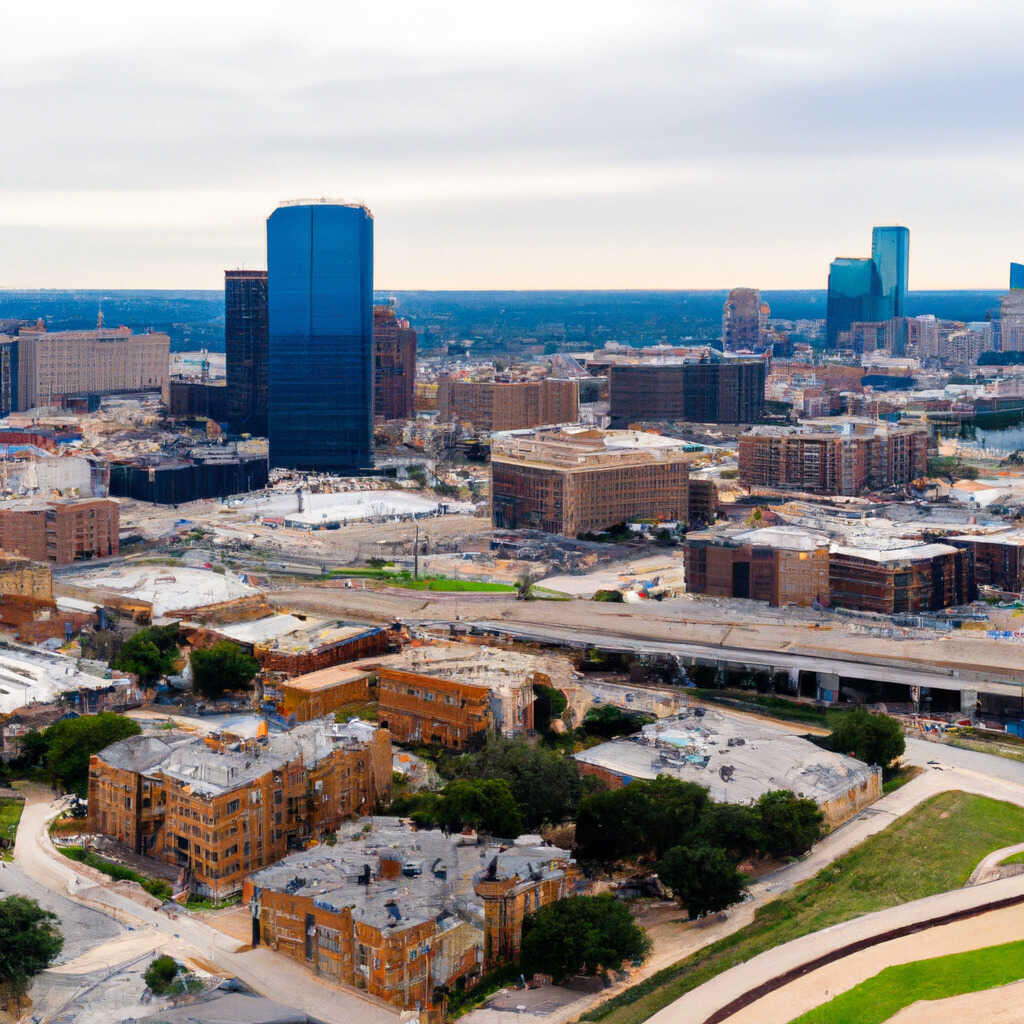This aerial photograph depicts a small city skyline characterized by a mix of mid-rise and high-rise structures. Dominating the bottom center are five to seven-story buildings made of orange brick with gray rooftops, likely residential apartments, surrounded by a network of roads. The bottom right features a green grassy area intersected by a walkway or roadway. The middle distance reveals an elevated highway stretching from right to left, cutting through the cityscape.

To the left, prominently, stands a towering, deep blue glass office tower, approximately 30 stories tall, accompanied by a darker office structure behind it and a substantial black building at its base. Adjacent to these is a much taller brown building, roughly half the height of the blue glass tower. Towards the top right, the skyline includes additional low-rise buildings and two more blue glass towers, one of which is taller than the other. The upper part of the photo features a hazy gray sky, adding a sense of depth to the cityscape.